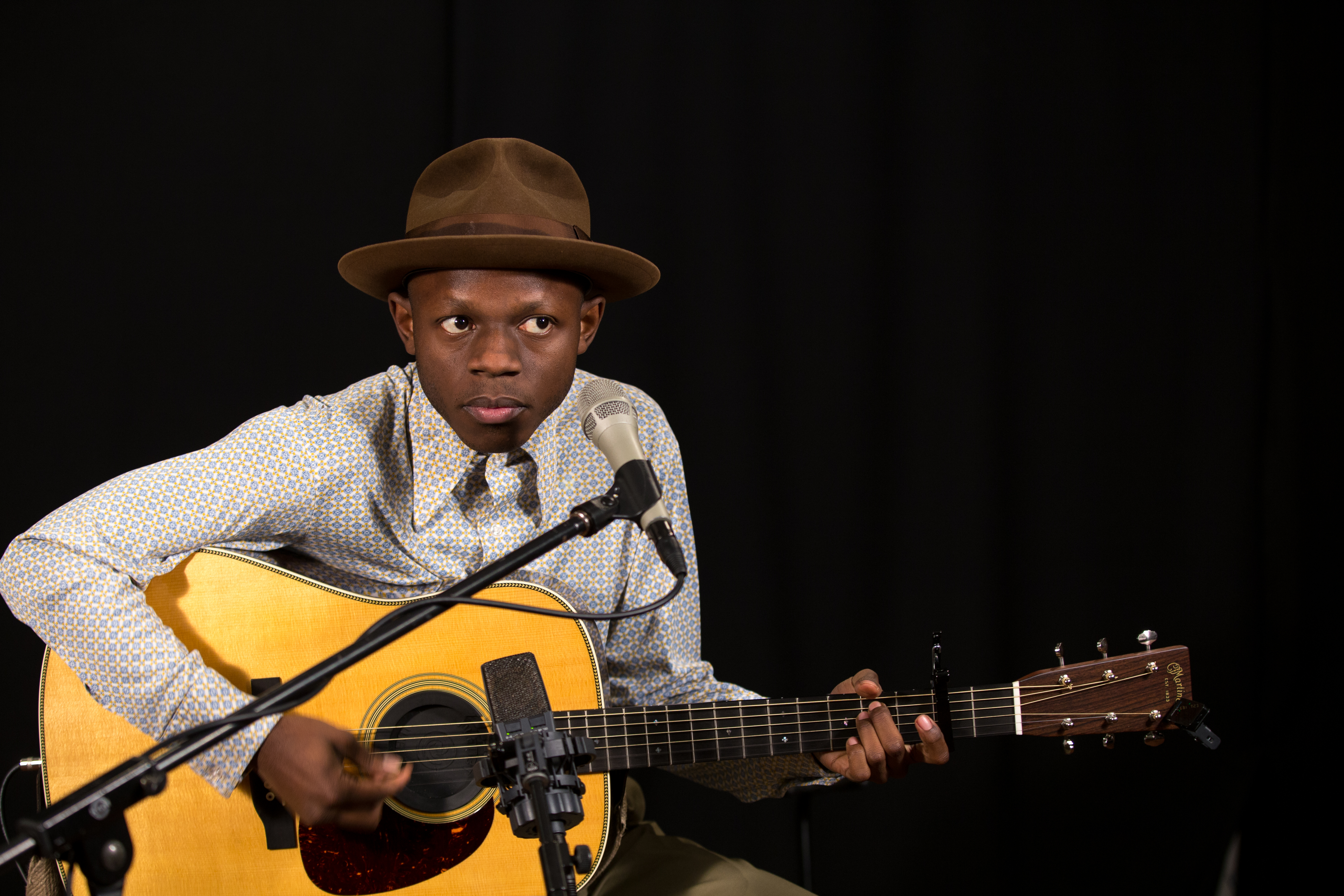In the image, an African American young man is seated and holding a guitar, positioned slightly left of center against a predominantly black background that resembles a curtain, suggesting an indoor setting, possibly during a music concert. He is facing forward, with his eyes looking to the right, and he's wearing a brown bowler hat and a white collared long-sleeve shirt with blue speckled designs. His right hand is strumming the guitar while his left hand is on the chords. A long black microphone stand extends from the bottom left corner of the image up to the right, with a silver microphone attached and directed toward his face. Additionally, there appears to be another microphone positioned just left of center, coming up from the bottom of the image and partially blocking the guitar. His tan-colored pants are partially visible under the guitar. The colors present include black, brown, white, blue, yellow, tan, and silver, and there is no text visible in the image.